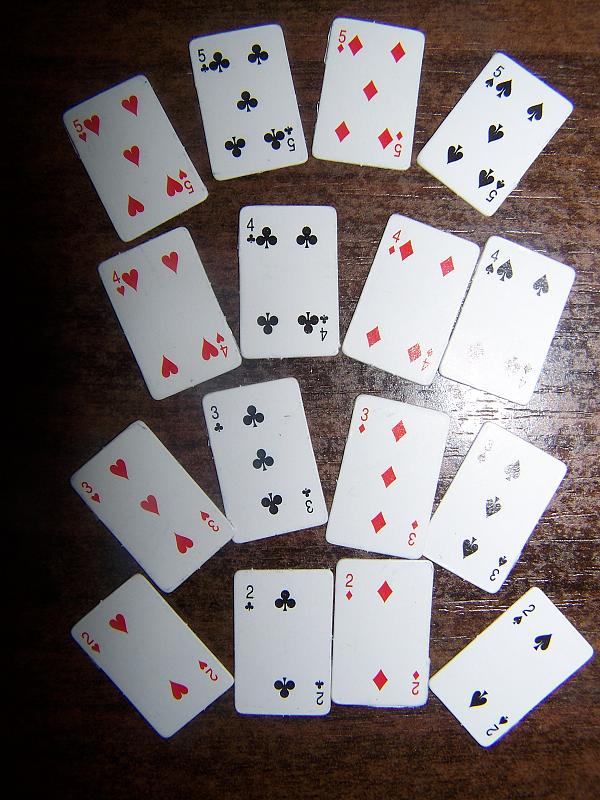The photograph showcases a meticulously arranged deck of playing cards spread across a wooden table, illuminated from above. The lighting creates a noticeable reflection on the right side of both the tabletop and the cards. 

On the left side of the image, the Hearts suit is displayed in a vertical sequence, featuring the 5, 4, 3, and 2 of Hearts from top to bottom. Adjacent to these, the Clubs (referred to as Clovers) cards are similarly arranged in descending order with the 5, 4, 3, and 2 of Clubs. Continuing rightward, the Diamonds suit follows the same descending pattern, showcasing the 5, 4, 3, and 2 of Diamonds. 

The rightmost section of the table displays the Spades suit, also in descending order, with the 5, 4, 3, and 2 of Spades. 

Cards at the center of the photograph are positioned more vertically, while those on the left and right edges are fanned out, creating an aesthetically pleasing, symmetrical display that highlights the distinctiveness of each suit.